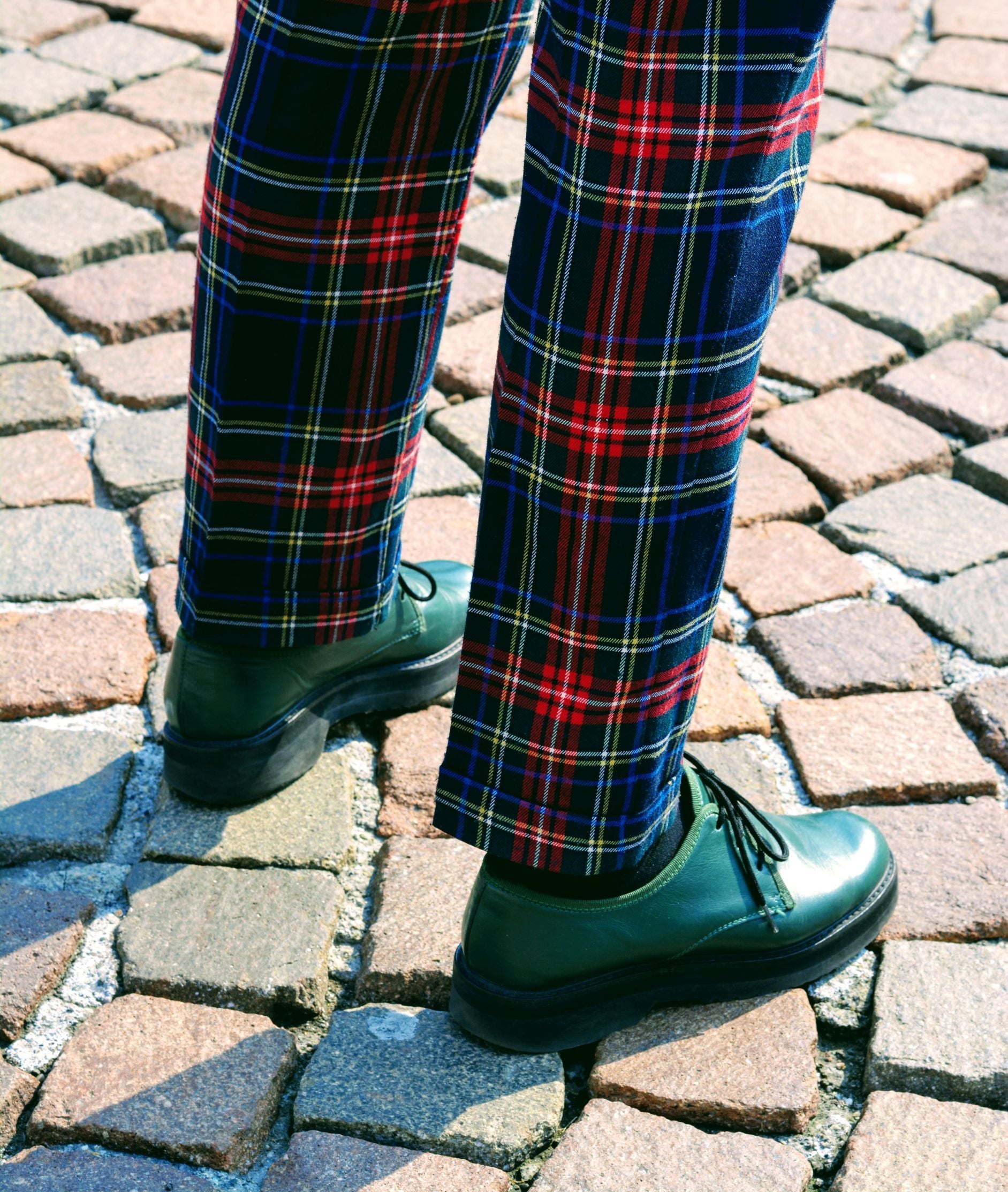A detailed image captures a person's neatly tied dark green loafers with black soles and black shoelaces, standing firmly on a cobblestone pathway. The shoes have a subtle bluish hue, complementing the person's vibrant plaid pants that feature intersecting stripes in red, various shades of blue, yellow, and darker hues at the intersections. The brick pathway beneath displays a mix of red and gray tones, with visible mortar in between, some of it worn away, hinting at the age of the bricks. The sun casts a shadow of the person's legs, emphasizing the textured contrast between the clean, well-maintained loafers and the weathered cobblestones.